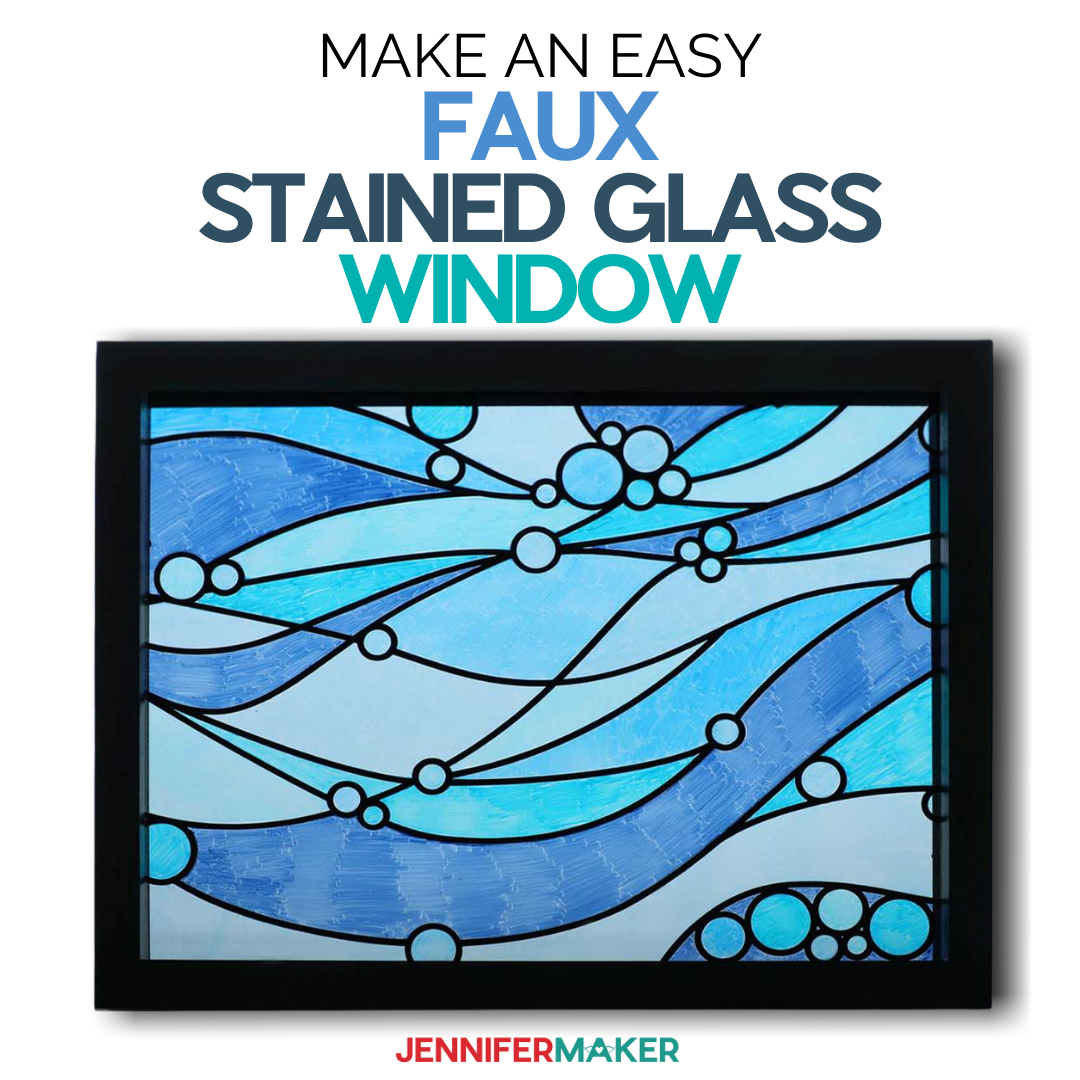The image features a horizontally framed piece of art resembling a stained glass window on a white background. The top section of the image displays the text "MAKE IT EASY" in thin black, all-caps font. Below that, "FAUX" is written in a bright blue color, followed by "STAINED GLASS" in a darker blue-green shade, and finally, "WINDOW" in a lighter green hue.

The centerpiece of the image is a stained glass artwork encased in a thick black frame. The design comprises an array of long, gently curving black lines that segment the piece into various shades of blue, ranging from turquoise and teal to dark navy and light grayish-blue. The lines and segments create a visual effect reminiscent of flowing water or ocean waves. Within the segments, small round balls in corresponding colors add a dynamic touch to the composition.

Beneath the stained glass artwork, the artist's name "JENNIFER MAKER" is prominently displayed. "JENNIFER" is in a bold reddish-pink color, while "MAKER" is in a blue-green shade, featuring a small heart within the letter "A" instead of a standard space.

The meticulous color variances and black line separations evoke the textures and fluidity of flowing water, lending the artwork a serene, oceanic feel.